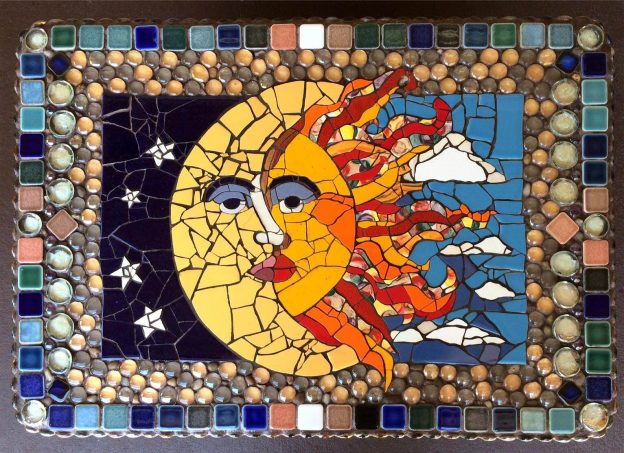This image showcases a captivating mosaic art piece featuring an intermingling sun and crescent moon. The composition forms a complete face with a shared set of eyes, nose, and mouth. The left half, representing the crescent moon, is set against a dark blue background adorned with white stars. The right half, representing the sun, is depicted with bright red lips and is set against a light blue sky with white clouds. The sun's rays stretch outward to the right, while the moon's natural-colored lips add subtle contrast. The mosaic is framed with circular decorative patterns of smaller pebbles transitioning to larger ones, all bordered by squared tiles. A dark blue border cleanly encapsulates this harmonious celestial interaction.